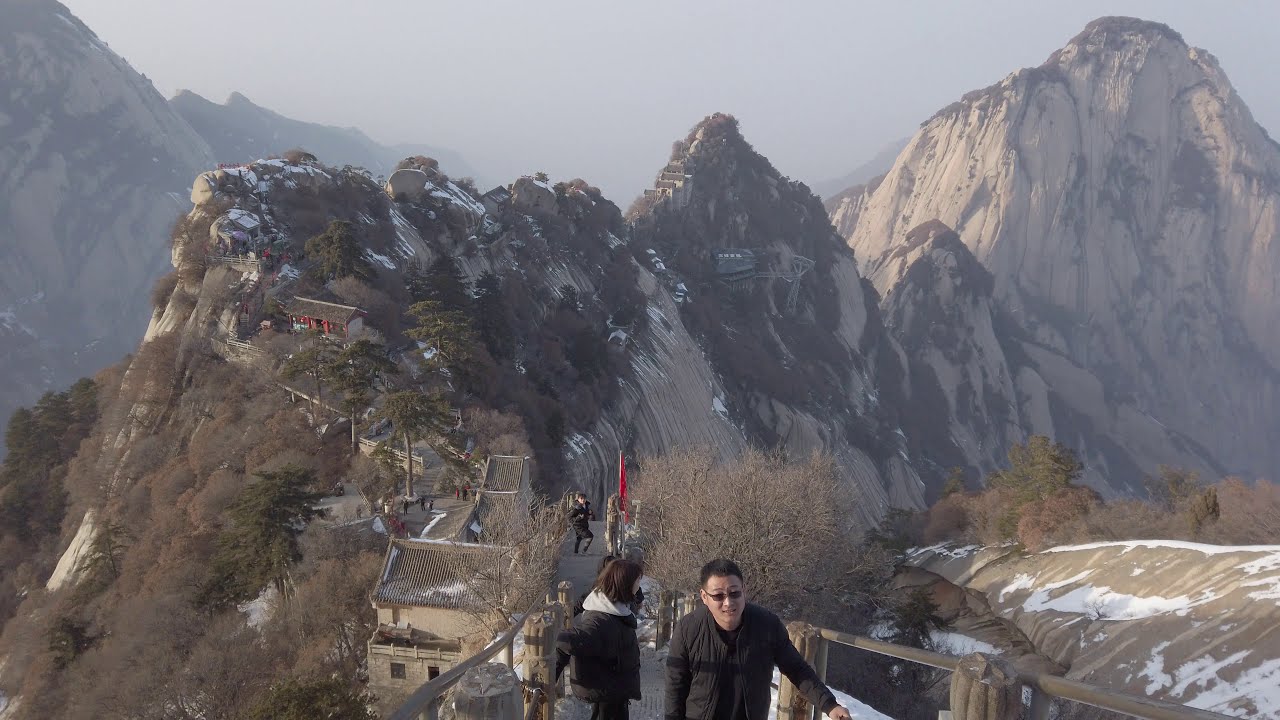The photograph captures a scenic mountain area viewed from a high elevation, with the focal point being a pathway bordered by railings. In the foreground, two individuals are walking along this path; one appears to be an Asian man with sunglasses and short black hair, dressed in a black sweatshirt, who is looking towards the camera. Beside him, a woman with shoulder-length dark hair, clad in a black jacket, is gazing off to the left. Further back on the path, another person can be seen, possibly on a small bridge. The background reveals a majestic mountain range with patches of snow and areas of bare, brown terrain dotted with green scrub brush. The sky above is overcast, adding a misty atmosphere to the scene. Snow can also be seen in the foreground to the right, hinting at the cold conditions suggested by the warm clothing of the people.